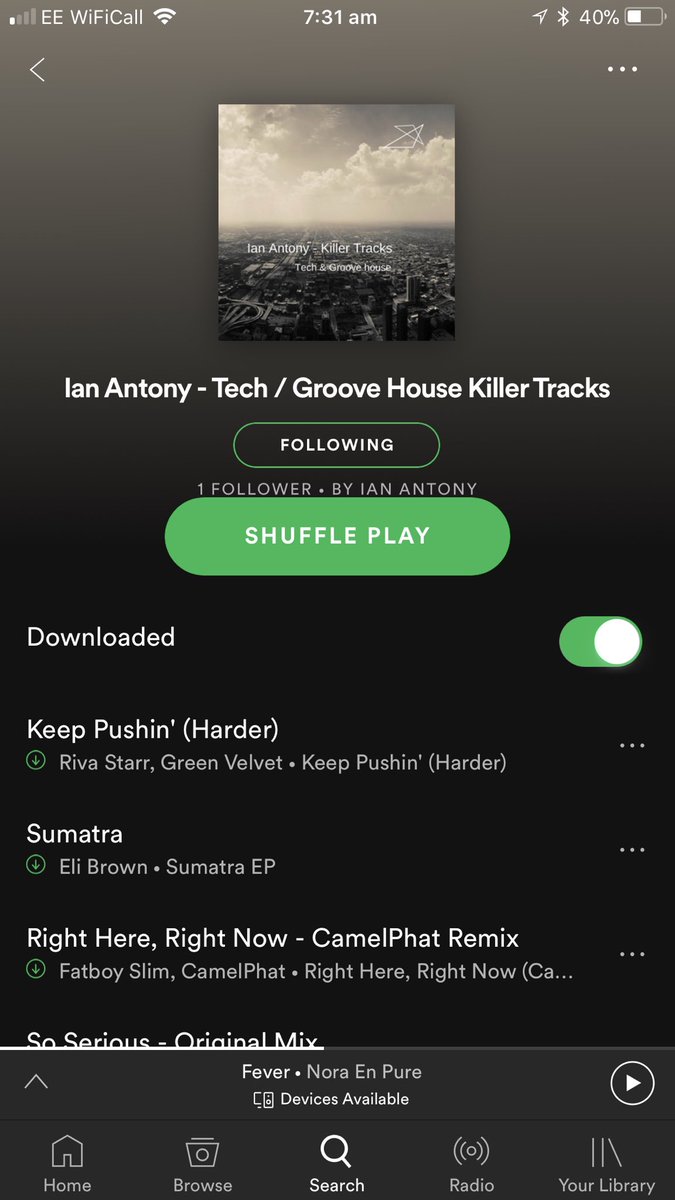Screenshot of a music playlist on a mobile device. The top of the screen displays various status icons on a gradient gray background. Starting from the left, it shows full Wi-Fi signal strength, the label "EE Wi-Fi Call," the time "7:31 AM" in the center, and in the upper right-hand corner, there are the battery percentage, Bluetooth logo, and the location icon.

The open playlist features the currently playing track: "Tech/Groove House Killer Tracks" by Ian Anthony. Below this, there is an indicator showing that the user is following this band. The "Shuffle Play" button is prominently displayed in green with white text. Below that, the word "Downloaded" appears on the left-hand side beside a toggle switch that allows the user to manage downloaded items.

The playlist includes the following tracks:

1. "Keep Pushin' Harder" by Riva Starr, featuring Green Velvet
2. "Sumantra" by Eli Brown, from the "Sumantra EP"
3. "Right Here, Right Now (CamelPhat Remix)" by Fatboy Slim, remixed by CamelPhat